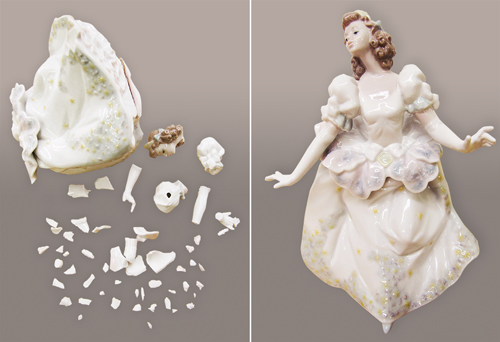The image is a horizontal rectangle divided into two sections, each containing a black and white photograph. The left side shows a broken porcelain doll, fragmented into numerous pieces scattered on a light gray surface. The larger intact pieces include parts of the dress and the doll's head, which features blonde curly hair with a bow. Among the tiny fragments, an arm and a hand are discernible. The right side of the image displays the fully assembled doll, now pieced back together. The doll, resembling a ballerina, stands with arms outstretched and fingers slightly open, creating a delicate pose. She wears a large, fancy dress with poofy sleeves that taper into elastic cuffs and then expand again in ruffled poofiness. The dress is low-cut and fitted down to the waist before blossoming out like a flower petal, ending in a wide, lace-trimmed skirt that fans out around her feet, featuring a pointed toe. The doll's expression is serene, with her head turned slightly to the side, showcasing her detailed face and flowing hair.